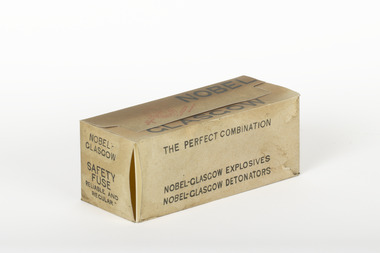The image depicts a rectangular, cuboid-shaped cardboard box positioned diagonally with its top higher on the right and lower on the left. The box, tan or light brown in color, appears slightly open at one corner. It has black text on all its visible surfaces: the longer side reads "The perfect combination, Noble Glasgow Explosives, Noble Glasgow Detonators," while the shorter, left face is inscribed with "Noble Glasgow Safety Fuse." The top of the box shows the text "Noble Glasgow." The photograph is set against a plain, light beige background, highlighting the simplicity and utilitarian design of the package, suggestive of its contents related to explosives.